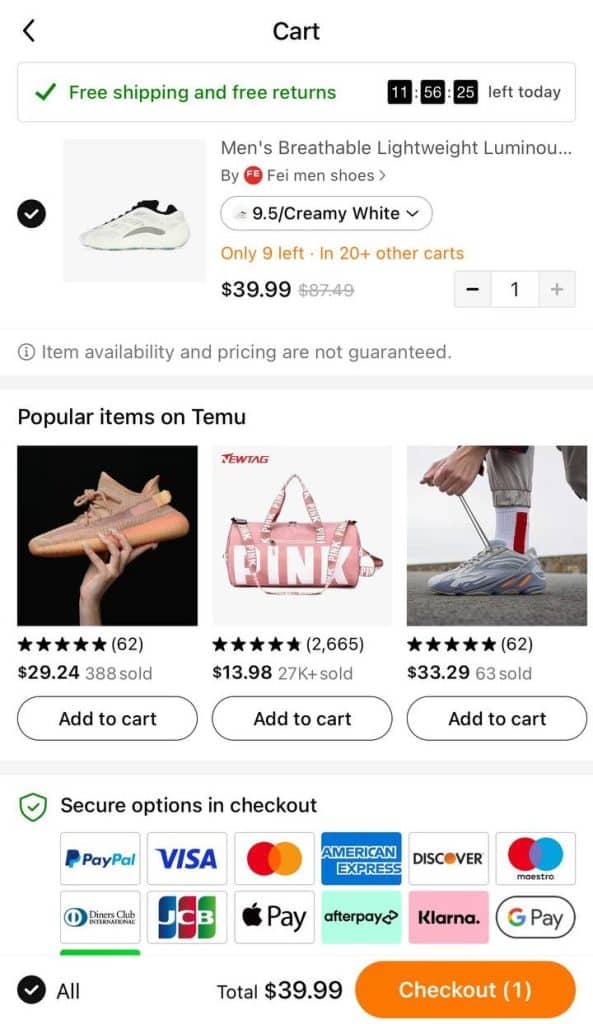The image displays the Teemo app interface on a mobile device, focusing on the cart section. The background is a clean white, ensuring clarity. At the top of the screen, the word "Cart" is prominently displayed, accompanied by a banner offering "Free Shipping and Free Returns." A countdown timer shows "11 hours, 56 minutes, and 25 seconds left" for the offer.

The cart contains a single item: "Men's Breathable Lightweight Sneakers," priced at $39.99, which is prominently displayed. Beneath the item description, a disclaimer notes that "Item availability and pricing are not guaranteed."

The lower portion of the screen highlights popular items on Teemo with images including a sneaker, a duffel bag, and another pair of shoes. Below this section, various secure payment options are presented for the user's convenience.

At the bottom of the screen, the total cost of $39.99 is visible, along with an orange "Checkout" button, urging the user to finalize their purchase. The original price of the sneakers, $87.49, is also indicated, emphasizing the current sale price of $39.99.